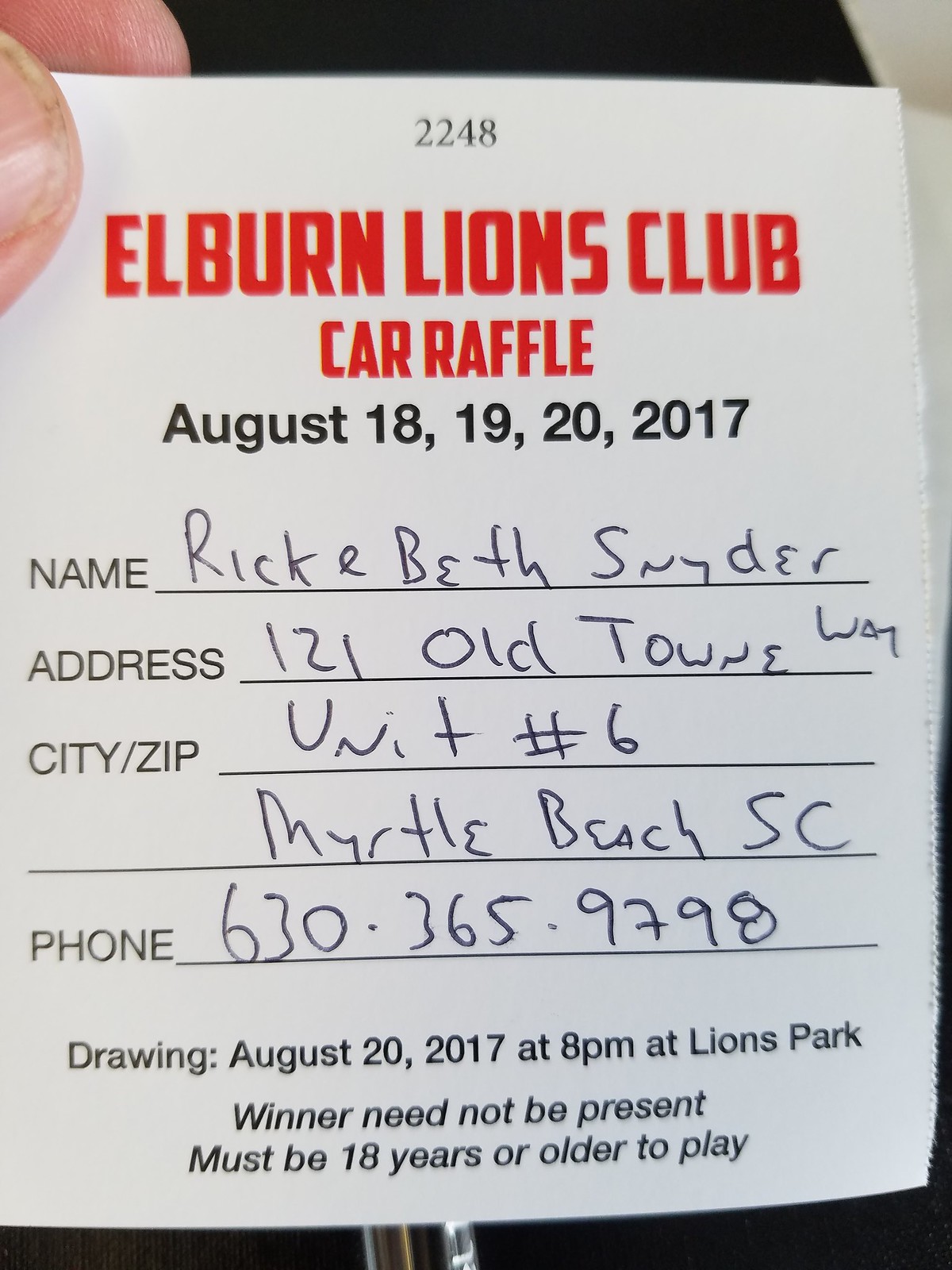The image depicts a raffle ticket for the Elburn Lions Club car raffle, held against a red and white background. The top of the ticket features the number "2248" printed in black. Beneath this, bold red text announces "Elburn Lions Club Car Raffle," followed by black text with the event dates, "August 18, 19, 20, 2017." 

The central section of the ticket includes spaces for personal information: name, address, city, zip code, and phone number. These lines have been filled out in pen with the name Ricky Beth Snyder, address 121 Old Town Way, Unit Number 6, Myrtle Beach, SC 63036, and phone number 597-9798. 

At the bottom of the ticket is the drawing information in black print: "Drawing August 20th, 2017 at 8 p.m. at Lions Park. Winner need not be present. Must be 18 years or older to play." 

The upper left corner of the image shows two fingers, one with a dirty fingernail, holding the ticket.